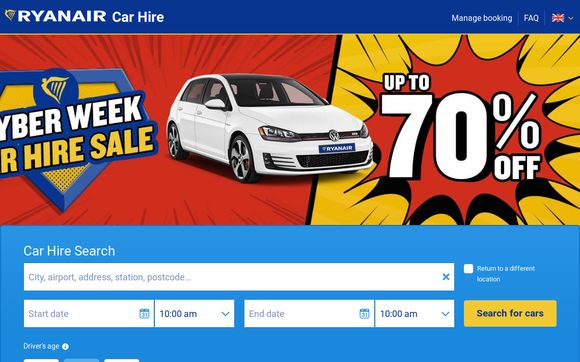The image showcases a Ryanair webpage with distinct sections and elements. At the top of the page, there is a dark blue header featuring the white text "Ryanair" alongside their logo on the left. To the right of the header, there are options for "Car Hire," "Manage Booking," "FAQ," and a British flag with a dropdown menu next to it.

In the middle of the page, a prominent graphic is displayed, split into two contrasting backgrounds. The left side has a red background with a blue and yellow logo along with the text "Cyber Week Car Hire Sale" and an image of a white hatchback car. The right side has a yellow background featuring a red splotch advertising "Up to 70% Off" in white text.

At the bottom of the page, there is a light blue rectangular box that spans the width of the page, labeled "Car Hire Search" in white text. This section includes several input fields: 
- A text box for "City, airport, address, station, postcode."
- A calendar selection box for the "Start Date" along with a dropdown menu for the time. 
- Another calendar selection box for the "End Date" with a corresponding dropdown menu for the time.
To the right of these input fields, there is a yellow button with blue text that reads "Search for Cars."